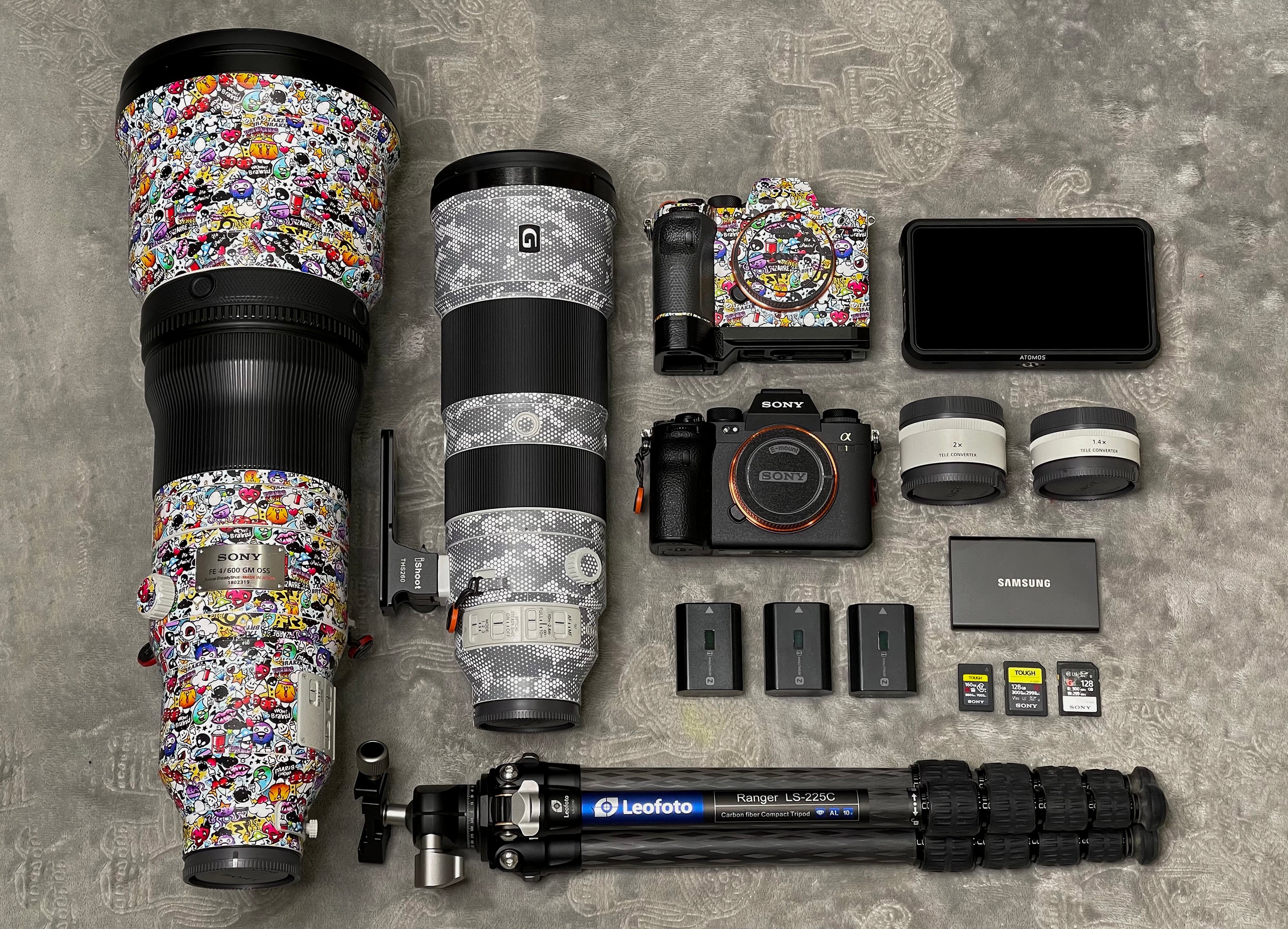This photograph features an organized array of camera and telescope equipment set against a gray, textured surface that varies in tones from light gray to taupe. Dominating the left side of the image is a large, cylindrical piece resembling a camera lens or telescope scope, decorated with a colorful, cartoonish pattern of smiling faces and various lively imagery. This piece is the largest component, standing erect and shaped like a flashlight, narrower at the bottom and widening at the top. Nearby, there's a slightly smaller lens featuring a gray camouflage motif, maintaining a similar vertical structure but in varying shades of gray.

In the upper right corner, there's a multicolored battery that might attach to the camera. Nestled in the center of the arrangement is a sleek, black Sony camera, prominently displaying the Sony logo on the center and top. To the right of this camera are two small lens attachments. Another Sony camera sits above the black one, distinguished by its vibrant, multicolored decal resembling a "Where’s Waldo" theme, covering most of its surface except for the grip area.

A horizontal, black tripod lies at the bottom of the photo, branded with "Leofoto Ranger LS-225C" and a blue and white logo featuring a leaf and camera icon. Additionally, the scene includes three small batteries that seem compatible with the Sony cameras, multiple memory cards, and a black box, possibly another camera, situated at the far right. These elements collectively illustrate a well-outfitted camera setup, ready for both artistic and technical use.